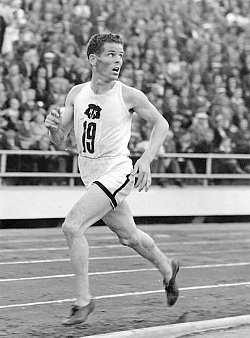This old black and white photograph captures a moment from a mid-20th century track and field event. The focus is on a male runner wearing vintage black running spikes without socks, racing on a dirt track. The stands are packed with a large, eager crowd, indicative of a significant event, possibly the Olympics, though the specific occasion remains unclear. The runner sports a white singlet and matching shorts, accented with black piping along the bottom and the sides. Pinned prominently to the front of his singlet is the number "19."

He has short, curly, blondish-brown hair, and his mouth is open as he glances over his left shoulder, perhaps checking a time display or responding to something happening off-frame. His attire features an unspecified logo on his chest, which may represent a country or organization. The runner appears to be mid-race, likely in a longer distance event such as a mile or half-mile, given his relaxed posture and attention to his surroundings. The historical ambiance of the photograph vividly evokes the athletic fervor and spectator enthusiasm of the era.